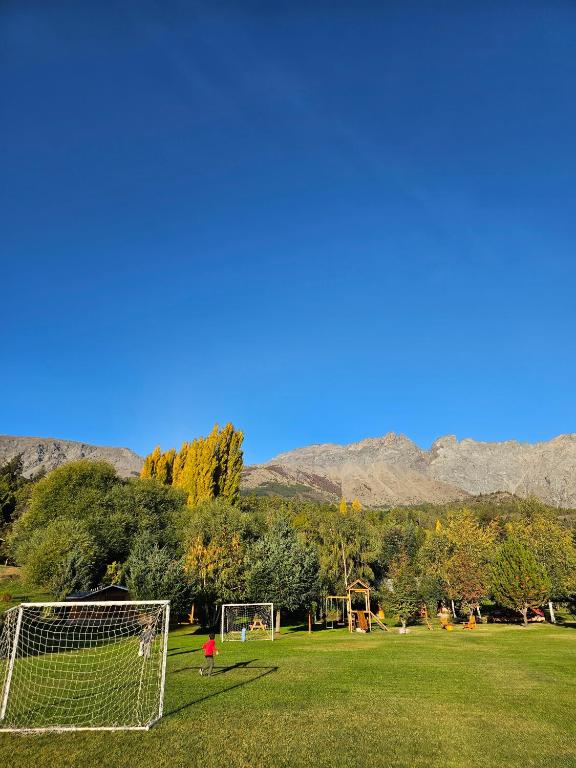This photograph captures a picturesque multi-purpose recreational area on a clear, cloudless day. The upper half of the image is dominated by a vast, gradient blue sky, transitioning from a deep blue at the top to a lighter blue as it meets a distant mountain range. In the middle ground, a diverse array of trees showcases an assortment of greens, from deep and bluish greens to yellowish hues. Below these trees, a lush green soccer field occupies the center, featuring two white nets. A child in a bright red shirt stands out vividly near one of the nets. To the bottom left, another net marks the other end of the field. The grass varies in its vibrant green color, with some patches turning grayish as they start to dry out. The edge of the tree line reveals a jungle gym, indicating the area is designed for various recreational activities. In the background, although difficult to see clearly, other children appear to be engaged in play. The scene perfectly blends the elements of nature and recreation, making it a visually appealing and dynamic photograph.